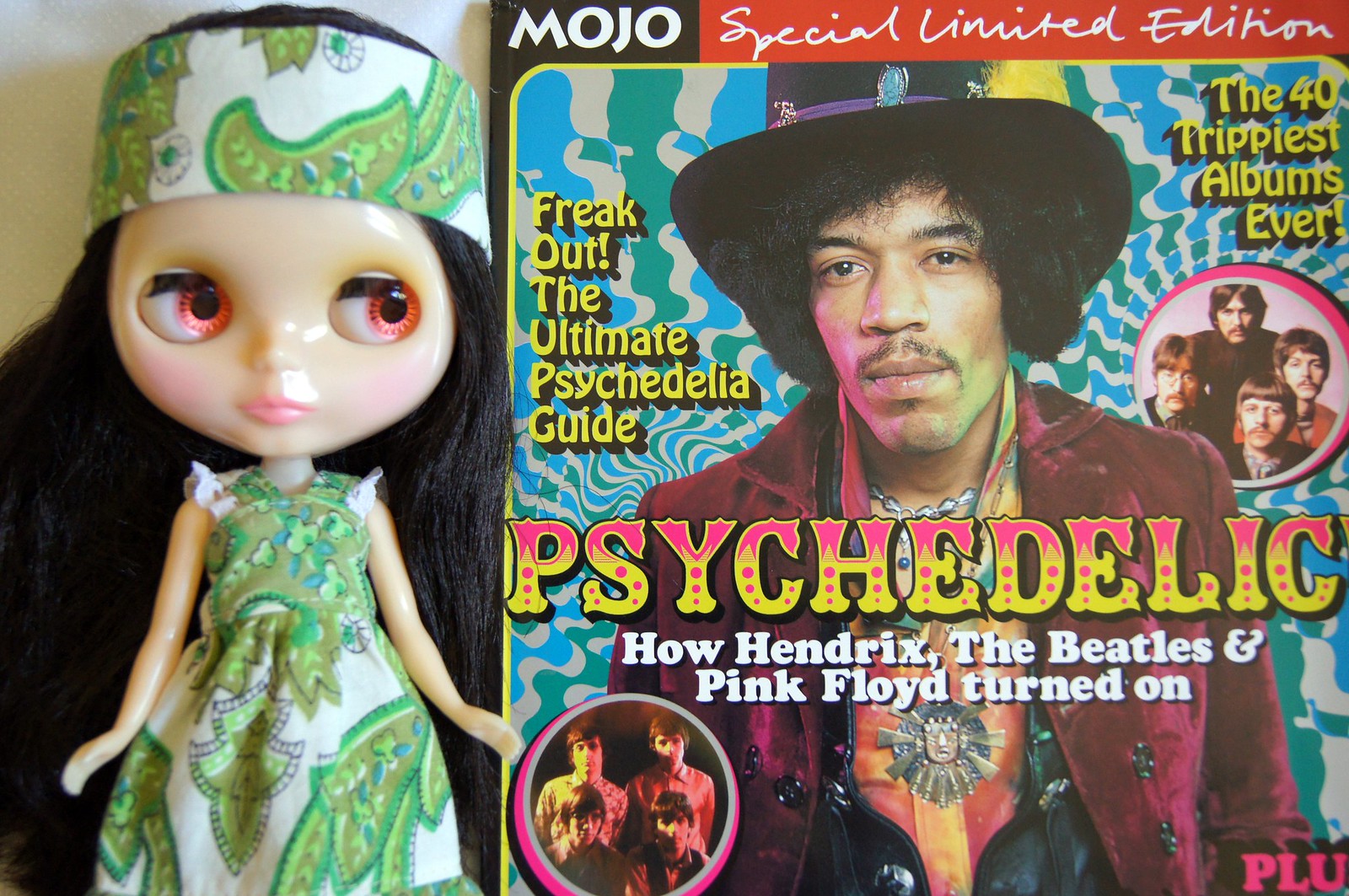The image features a striking magazine cover on the right, titled "Mojo Special Limited Edition." Centered on the cover is an iconic photograph of Jimi Hendrix, distinguished by his black hat adorned with a green or yellow feather, medium-length black hair, small mustache, maroon velvet jacket, red and yellow shirt, and black vest. Across Hendrix's chest, in bold pink and yellow letters, is the word "Psychedelic," with the subheading "How Hendrix, The Beatles, and Pink Floyd Turned On" in white text below. The content promises a feature titled "Freak Out! The Ultimate Psychedelic Guide" in yellow script, and in the upper right corner, it highlights "The 40 Trippiest Albums Ever."

To the left of the magazine cover stands a doll reminiscent of a Bratz doll, characterized by a large head and prominent pink eyes that gaze toward the magazine. The doll has long black hair and is dressed in a matching green and white patterned dress and headband, embodying a 1960s style. This doll adds a quirky touch to the image, its vibrant attire harmonizing with the psychedelic theme of the magazine cover. The image is rich with colors, predominantly featuring reds, yellows, and greens, which vividly evoke the spirit of the era depicted.